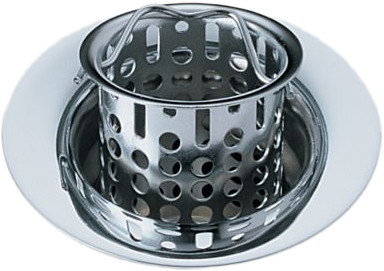The image showcases a product photo of a shiny, chrome-like drain stopper designed for sinks or bathtubs. The background is white, emphasizing the silver, reflective appearance of the device. It features a circular, curved outer rim that fits snugly into the drain opening. Extending downward from the rim is a cylindrical metal basket with a series of holes punched through it, varying between circular and oblong shapes. These holes are intended to allow water to pass through while trapping debris like hair or food particles, preventing them from clogging the pipes. A piece of bent metal wire is attached to the basket, providing a handle for easy removal and cleaning. The simplicity and functionality of this design highlight its utility in keeping drains clear.